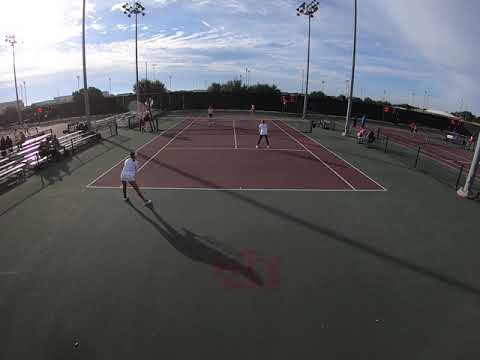The outdoor image captures a dynamic scene of a tennis or pickleball game in action, viewed from a slightly overhead angle. Four female players, dressed in white, are engaged in a match on a vibrant playing field. They are evenly split with two players on each side—one positioned near the net and their partner stationed towards the back of the court. The court itself features a striking color palette with a green outer field and a red playing area, all marked by crisp white lines.

Surrounding the court are lush palm trees and other distant foliage, framing the scene with natural beauty. The vibrant blue sky is dotted with numerous white clouds, contributing to the bright, natural daylight illuminating the game. On the left side of the image, there are bleachers that are sparsely populated, indicating a small audience watching the match. The overall clarity of the photo is quite good, offering a clear and detailed view of the sporting action and its picturesque outdoor setting.